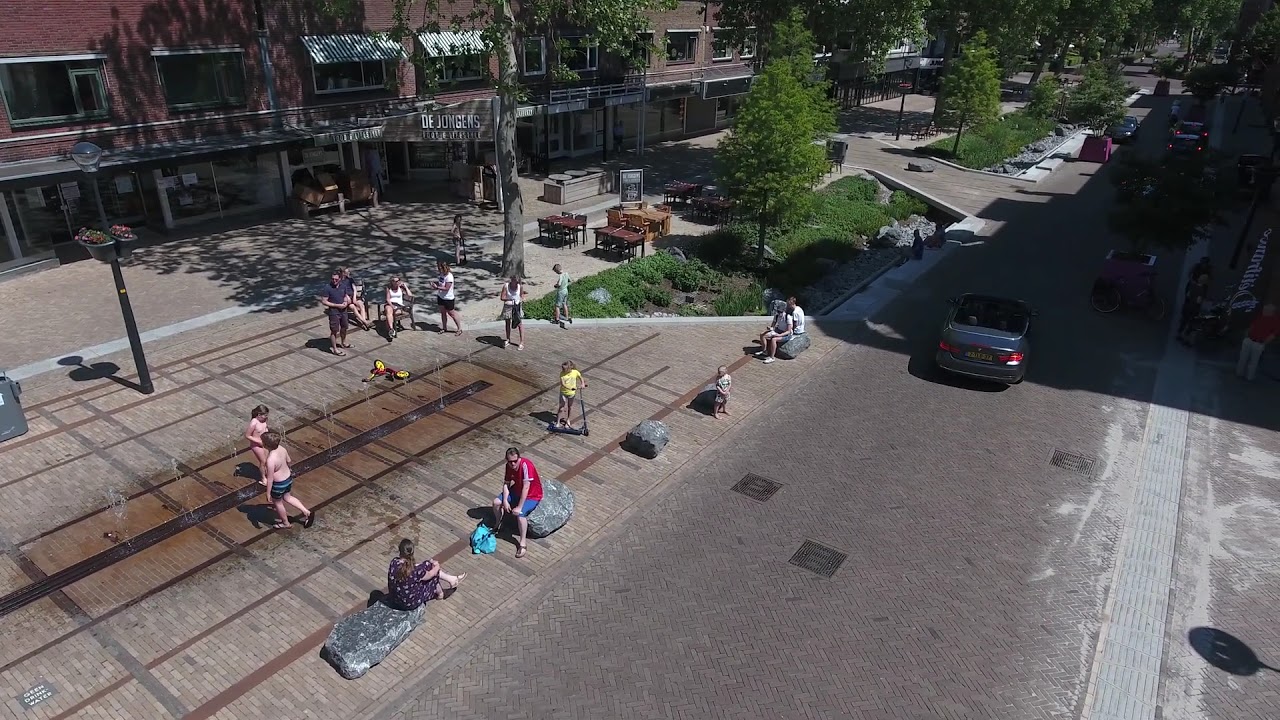The image, captured from an elevated perspective, showcases a bustling suburban street scene on a bright, sunny day. The wide roadway, lined with cars, runs parallel to a spacious, brick-paved sidewalk area where a simple splash pad with water jets shooting from the ground entertains children. Nearby, large rocks serve as casual seating for adults, who watch over the kids playing in the water. A little girl rides her scooter near the splash pad, adding to the lively atmosphere.

Adjacent to this playful scene, a row of uniform, at least two-story buildings, possibly housing shops and stores, extends along the street. A patio with wooden furniture suggests a café or restaurant space where people can relax. In the background, leafy trees frame the scene, adding a touch of greenery. Notably, a sign in the upper right-hand corner casts a shadow, while another sign, bearing the name "Dejongans," is visible on a large building in the top left-hand corner. The image is bright and clear, illuminated by natural sunlight, capturing the essence of a community enjoying a warm day.